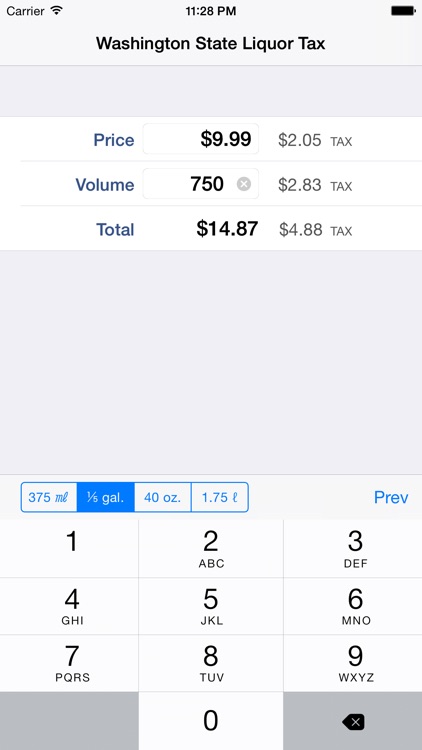This is a detailed caption of an image that depicts a mobile application interface displaying liquor tax information in Washington State.

---

The photographic image captures a mobile application interface on a phone screen. At the top right of the screen, the carrier signal is indicated with three out of four bars, and the Wi-Fi strength is also shown with full bars. The time displayed on the phone is 11:28 PM, and the battery icon shows it is fully charged, all rendered in black.

Dominating the upper section of the screen is the heading "Washington State Liquor Tax" in bold, black font. Just below, you see detailed pricing information:
- The price for an unspecified item is listed as $9.99, with an additional tax of $2.05 shown in gray text. The price itself is highlighted in blue.
- Another item is listed with a volume of 750 milliliters, priced at $7.50 with a tax of $2.83, again with the price in blue.
- The total amount calculated is $14.87 with a total tax of $4.88 also displayed.

Towards the lower part of the screen, there is a calculator interface complete with digits from 1 to 0, providing interactive number input capability. A blue box highlights the volume of 375 milliliters, and next to it, "Half Gallon - 40 Ounces - 1.75 Liters" is displayed in bold.

At the very bottom, a blue button labeled "Previous" is visible. Some numbers on the interface appear grayed out, and a black back button is also present, presumably to navigate to the prior screen.

The overall design of the app is visually organized, with a blend of colors like blue, gray, and black to differentiate between various pieces of information.

---

This caption offers a comprehensive description of the mobile application's interface, emphasizing the layout, colors, and specific details displayed on the screen.